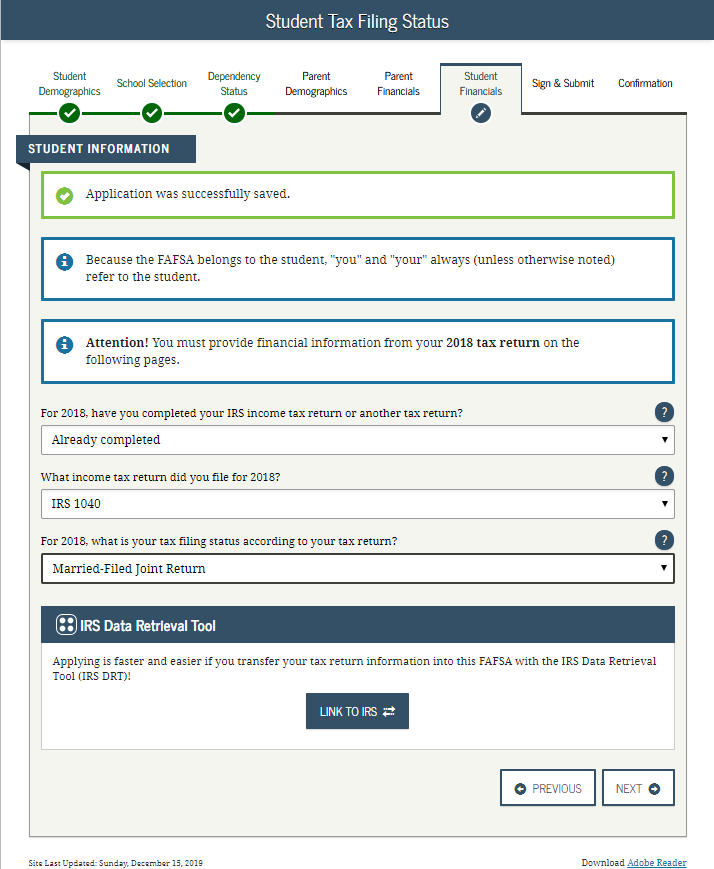In the image, we are looking at a screenshot taken from a tablet. The screenshot features a user interface with a dark blue header displaying white text that reads "Student Tax Filing Status." Below the header, there are a series of tabs aligned from left to right:

1. Student Demographics - Marked with a white checkmark inside a green circle.
2. School Selection - Also marked with a white checkmark inside a green circle.
3. Dependency Status - Similarly marked with a white checkmark inside a green circle.
4. Parent Demographics
5. Parent Financials
6. Student Financials - This tab is currently open and marked with a white checkmark inside a green circle.
7. Sign and Submit
8. Confirmation

Within the open "Student Financials" tab, there is a message that reads: "Application was successfully saved." Beneath this message, additional text states: "Because the FAFSA belongs to the student, 'you' and 'your' always, unless otherwise noted, refer to the student. Attention: You must provide financial information from your 2018 tax return on the following pages."